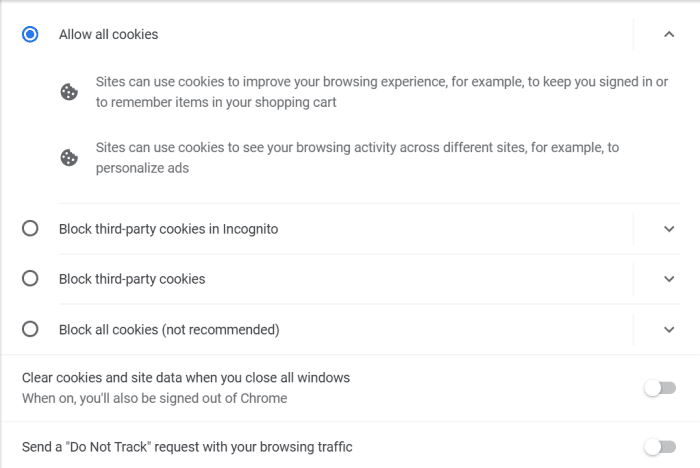**Descriptive Caption:**

The screenshot captures a browser's cookies settings menu, displayed on a clean white background. At the top of the menu, a blue radio button is ticked next to the option "Allow all cookies," indicating this preference is currently selected. Below this, a subsection elaborates with two bullet points, each marked by a cookie icon. The first bullet point explains that "Sites can use cookies to improve your browsing experience, for example, to keep you signed in or remember items in your cart." The second states that "Sites can use cookies to see your browsing activity across different sites, for example, to personalize ads."

A thin separator line follows, leading to the next option, "Block third-party cookies in Incognito," accompanied by an unticked, empty radio button. Another thin line comes next, preceding a collapsed submenu titled "Block third-party cookies," which also has an unticked, white radio button.

Further down is the option "Block all cookies (not recommended)," again marked by an unticked radio button. This section has been expanded to reveal additional settings: "Clear cookies and site data when you close all windows," with a note that enabling this will sign you out of Chrome, and "Send a 'Do Not Track' request with your browsing traffic." Both of these options feature toggle switches on the right, neither of which have been activated, as indicated by their lack of color.